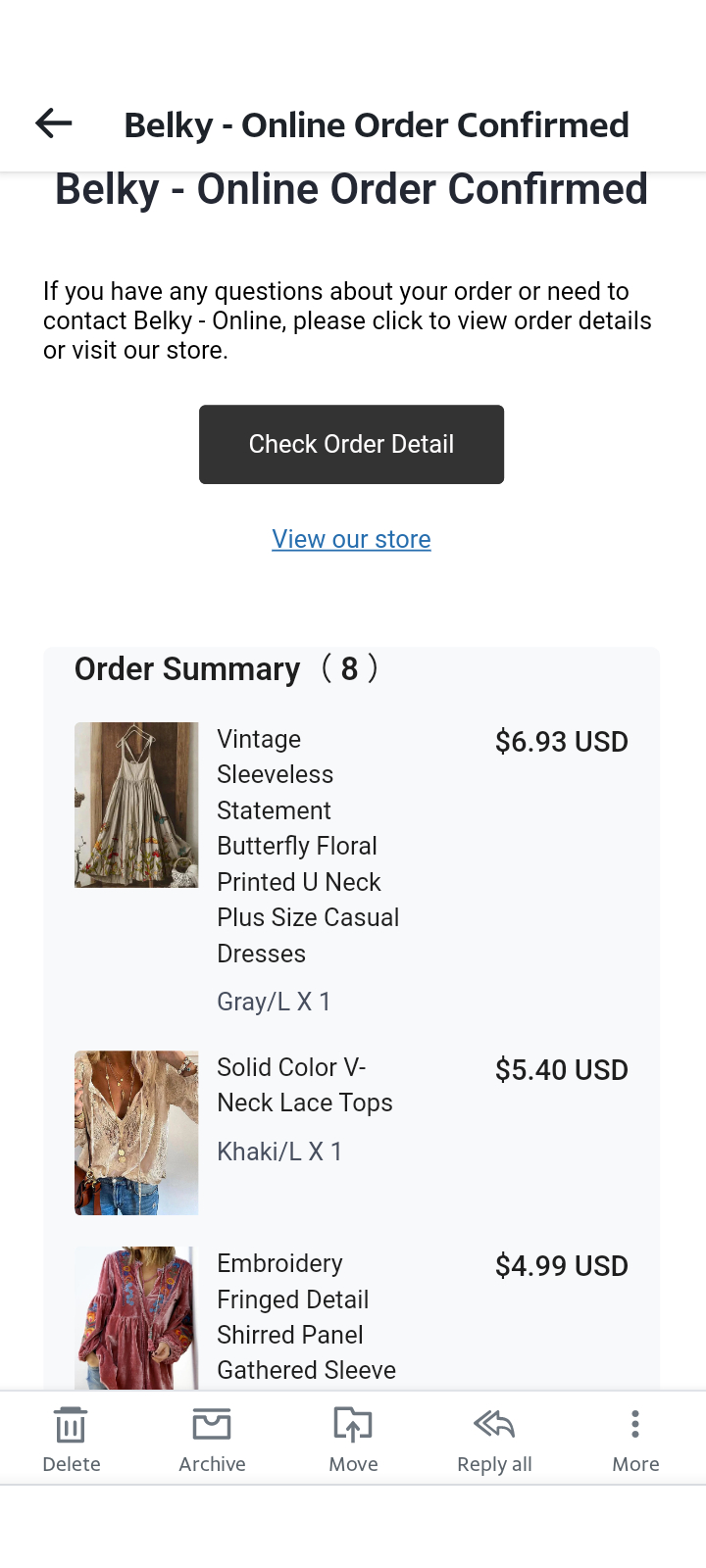The image depicts a phone application interface where a user is shopping for clothes. The screen confirms a Belki Online order, stating: "Online Order Confirmed. If you have any questions about your order or need to contact Belki Online, please click to view order details or visit our store."

Beneath this message is a prominent button labeled "Check Order Details," along with an option to "View Our Store." Below these options, an order summary is partially visible, showing details for 3 out of 8 pieces of clothing ordered.

1. The first item is a dress shown on a hanger, described as "Vintage Sleeveless Statement Butterfly Floral Printed Unite Plus Size Casual Dress, Gray, LX1" priced at $6.93 USD.
2. The second item is a white blouse, described as "Solid Color V-Neckline Tops, Khaki, LX1" priced at $5.40 USD.
3. The third item is a pink coral-colored shirt, described as "Embroidery Fringe Detail Shirt with Panel Gathered Sleeves" priced at $4.99 USD.

At the bottom of the screen, there are icons for various actions: "Detail," "Archive," "Move," "Reply All," and "More."